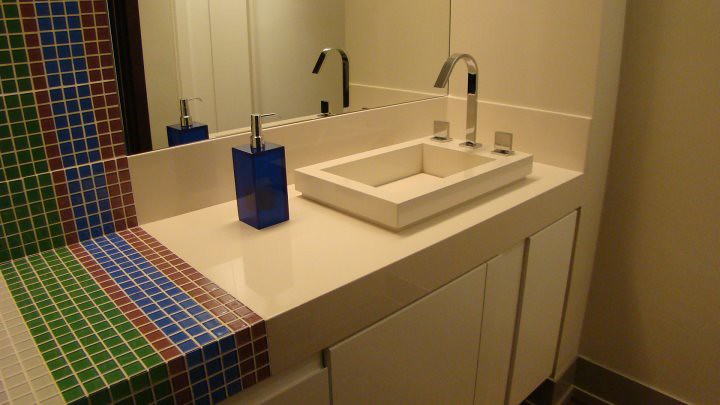The photograph captures a modern bathroom with an artistically tiled counter and wall. The counter, predominantly white, features intricate rows of small, colorful square tiles. These tiles are meticulously arranged in a pattern: two lines of brown tiles, followed by three lines of blue tiles, then a single line of brown tiles, and five lines of green tiles, concluding with three visible lines of white tiles. This design extends from the front edge of the counter, up and over to the back, continuing up the wall.

To the right of the counter, an expansive mirror occupies the remaining wall space, reflecting light and giving an illusion of a larger space. Below the mirror, the counter, sink, and surrounding cabinetry are all pristine white, contributing to a clean, cohesive look. The rectangular sink, characterized by sharp lines and silver fixtures, deviates from the norm with its faucet positioned on the right side instead of the traditional front placement. The faucet itself is flat, with a modern design featuring a curve that arches up and then down, accented by a black pad on its front. 

Practicality meets style with a tall, blue square soap bottle adorned with a silver pump, strategically placed to the left of the sink. The floor of the bathroom is trimmed with a dark brown border, grounding the light color scheme while adding a subtle contrast. This bathroom combines functionality with a touch of colorful elegance, showcased through its meticulously detailed design.